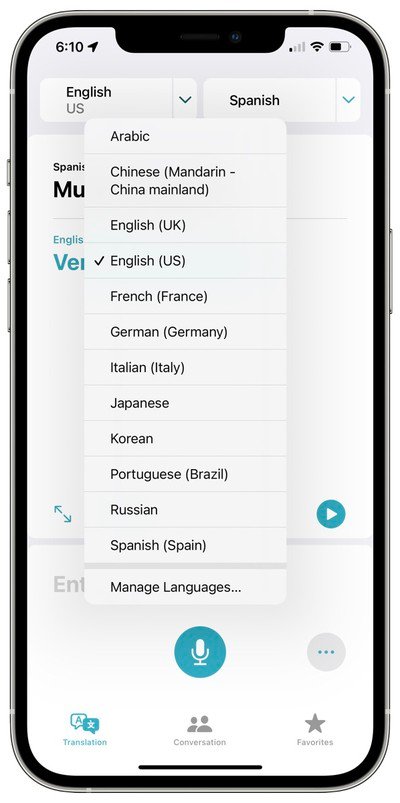The image depicts a smartphone featuring a sleek silver outline and a contrasting black front. On the left side of the device, three silver buttons are prominently visible, while the right side has a single silver button. The screen's background is primarily off-white, with a black section in the top-left corner displaying the time as "6:910" accompanied by the end of a black arrow pointing diagonally to the right.

The reception bar indicates poor signal strength with one black bar out of four, the remaining three being gray. Conversely, the Wi-Fi signal is strong, evidenced by a fully black icon. The battery indicator shows more than half of the battery life remaining.

On the left side of the screen, two boxes display the text "English" in black, with "U.S." underneath it in gray. A pop-up in the foreground is white, listing multiple languages. The first line reads "Arabic" in black text, followed by a thin gray line. Subsequent lines display "Chinese (Mandarin, China Mainland)," "English (UK)," "English (U.S.)," "French (France)," "German (Germany)," "Italian (Italy)," "Japanese," "Korean," "Portuguese (Brazil)," "Russian," and "Spanish (Spain)," each separated by thin gray lines. A thicker gray line follows, beneath which "Managed Languages" is written in black.